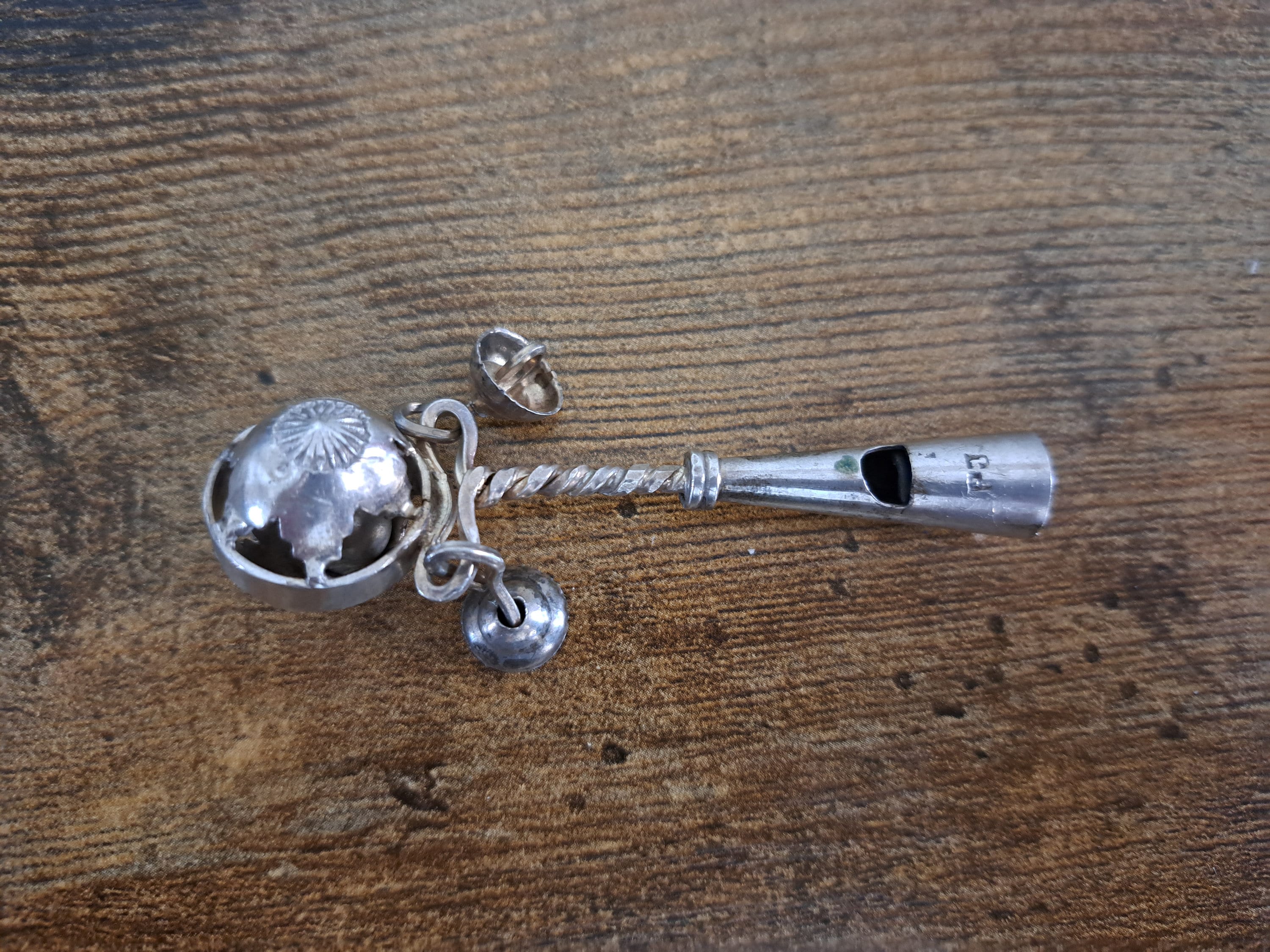The photograph, taken indoors, showcases a weathered dark brown wooden surface characterized by thin wavy horizontal lines and marked with scratches and indentations. At the very center of the image, a vintage silver-toned baby rattle and whistle rests prominently. The whistle, situated on the right-hand side, features a triangular shape with its wide base on the far right, narrowing as it extends leftward. This section, measuring just over an inch, includes an open area essential for sound production. Adjacent to the whistle, a twisted, corkscrew-like segment of metal spans about an inch, connecting to a small metal globe that forms the rattle’s chamber. This globe houses a rattle and is adorned with two bells suspended from either side of the twisted metal. One bell appears to be partially missing its underside. Notably, etched below the whistle is the marking "PJ," which may represent initials. The rustic wooden texture serves as a striking backdrop, enhancing the antique charm of this unique and intricate rattle and whistle.